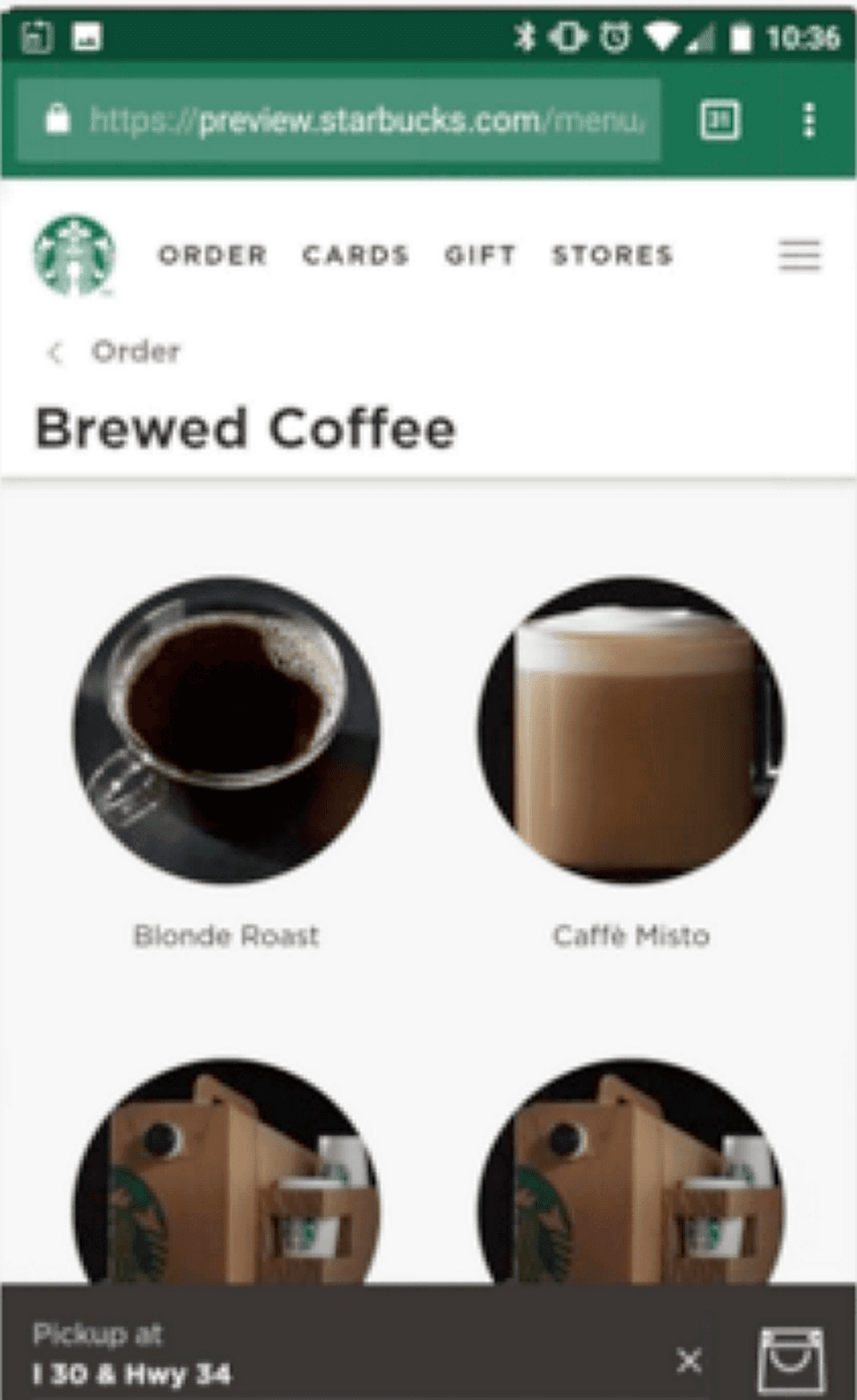This is a detailed screenshot of the order section in the Starbucks app. At the top of the screen is a green bar featuring a green search icon and the text "preview.starbucks.com/menu." To the right of this is a square tab icon displaying the number 35, indicating the open tabs.

Below the green bar, the page has a white background with the notable Starbucks logo situated at the top left. Next to the logo, there are several navigational categories listed in a horizontal line: "Order," "Cards," "Gift," and "Stores." To the far right of these categories is a menu icon.

Underneath this navigational bar, the word "Order" appears in small gray letters on the left side of the page, accompanied by a left-pointing arrow. Below this, "Brewed Coffee" is displayed prominently in large, bold black letters. Immediately under the "Brewed Coffee" title, there are four round image thumbnails presenting different coffee options. 

The top-left thumbnail features the "Blonde Roast," and the top-right thumbnail displays the "Caffè Misto." The titles of the bottom two thumbnails are truncated, but they depict to-go coffee containers, resembling group order boxes.

At the very bottom of the screen is a black banner. On the left side of this banner, the pickup location is displayed, while the far right side features an icon of a shopping bag.